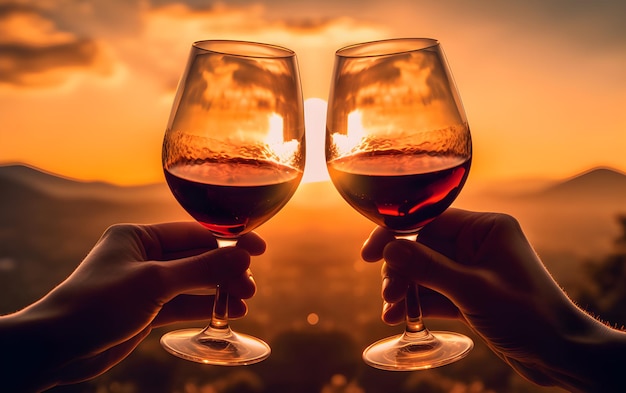The image captures a serene moment of celebration, showcasing the hands of two individuals each holding a clear wine glass, both containing about a quarter full of red wine. The glasses are held up and leaning towards each other, appearing as if they are about to clink in a toast. The setting sun in the background casts a warm, glowing light between the glasses, illuminating the scene with a beautiful light orange hue. The bottom half of the image is blurred with tones of brown and lighter orange, drawing focus to the vivid clarity of the toasting wine glasses against the picturesque backdrop. The overall image exudes an atmosphere of joy and the simple pleasure of sharing a moment at sunset.